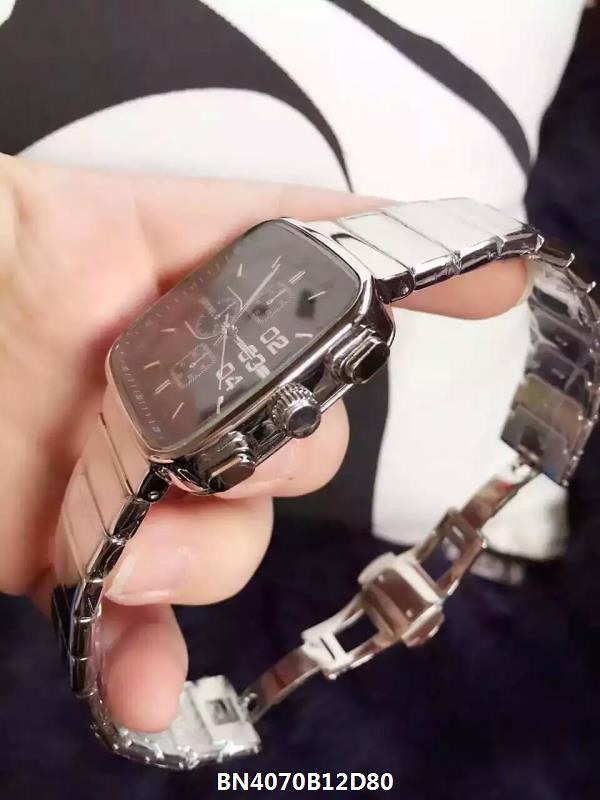This detailed photograph captures a close-up of a left Caucasian hand holding a silver watch. The watch is angled towards the upper left corner of the frame. The background features a white throw pillow adorned with black triangles, and beneath it, there appears to be a dark blue sheet. At the bottom of the image, the text "BN4070B12D80" is displayed in white font. The watch itself boasts a square face encased in a square silver bezel, accompanied by a silver chain band that is unclipped, revealing the clasp at the bottom. The watch face is predominantly black, embellished with white numerals or Roman numerals, and is complemented by silver hands. The watch case exhibits a notable shine, making the face of the watch partially obscured due to the reflective surface.